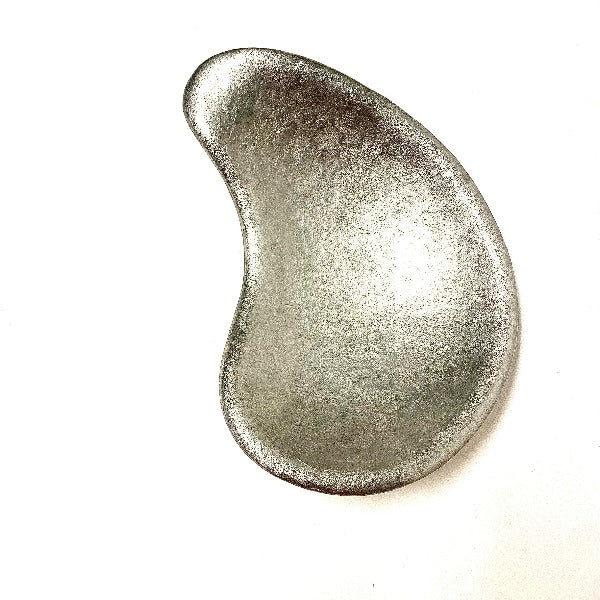The image depicts a close-up of a silver object with an indented, bowl-like depression, resembling a thumbprint. The object, primarily flat with a bulging, bean-like shape, is shaded in varying hues of grey, black, and white. Its surface reflects light, creating illuminated white patches, especially at the top, center, and along its outline. Darker grey and black areas accentuate its metallic texture. Positioned on a well-lit white-beige table, the object evokes the appearance of a slightly damaged pear due to its long, bulbous form. Despite uncertainty about its exact material, the object looks convincingly like a piece of metal.